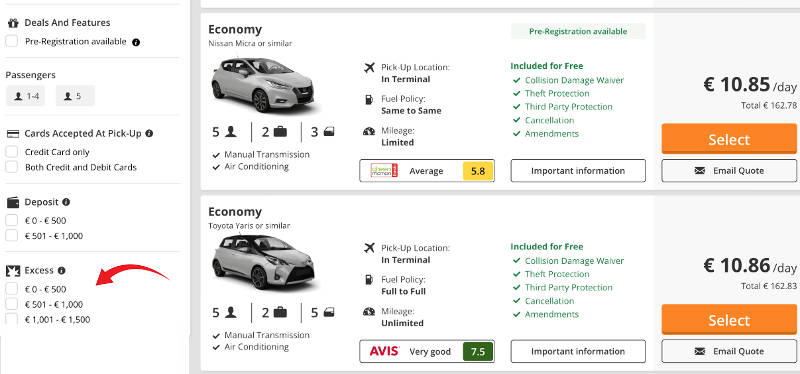The image showcases a rental car booking interface. On the left side of the screen are several filter criteria options, allowing users to specify their preferences for the rental car. Filters include the number of passengers the vehicle can accommodate, payment options (credit card or debit card), deposit amounts, and insurance excess options.

On the right side, the search results display two economy car options: a Nissan Micra and a Toyota Yaris. Each car listing provides detailed information about the vehicle's capacity, such as the number of passengers and luggage it can hold. Additional details include special features like manual transmission and air conditioning. The listings also specify pick-up locations, such as in-terminal options, fuel policies (limited vs. unlimited mileage), and pre-registration details.

A green list highlights complimentary inclusions such as theft protection, free cancellation, and booking amendments. The price per day for each vehicle is prominently displayed, along with an orange "Select" button for users to proceed with their booking.